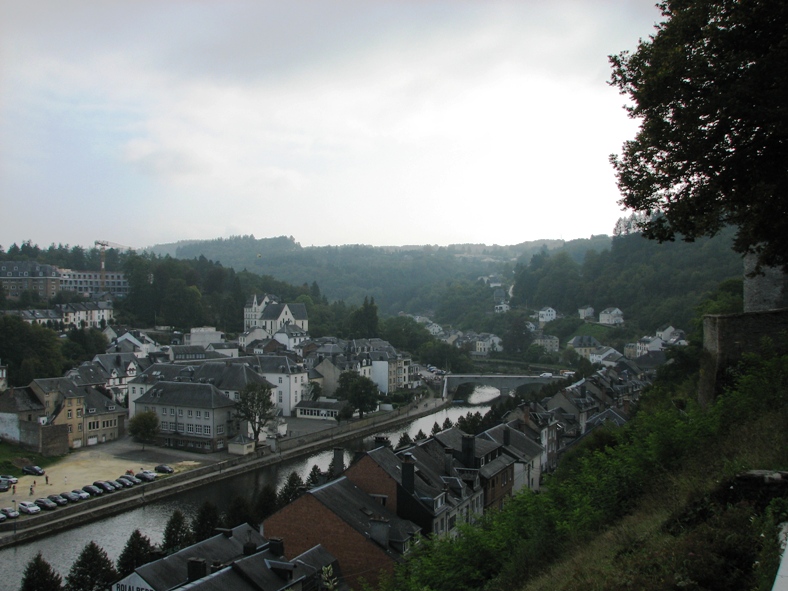The image is an overhead view of a quaint village nestled in a mountainous terrain. The scene is framed by a gray, cloudy sky with hints of blue visible in the upper right-hand corner. The landscape features lush green vegetation covering rolling hills and mountains in the distance.

In the center of the image, a river meanders through the village, flowing under a bridge before curving out of view to the left. On the right bank of the river, a line of houses with steeply pitched roofs and chimneys is visible, flanked by a row of green trees. On the left bank, a cluster of parked cars is seen facing the river, adjacent to several large buildings with steeply sloped roofs and numerous windows, some of which are two or three stories high.

Further up the hillsides and mountains beyond these buildings, even larger structures can be spotted. Scattered throughout the village are various other buildings, including businesses, creating a mix of architectural sizes and styles. A possible construction site, indicated by a small crane, can be observed on one of the hills.

The overall atmosphere of the village is busy yet orderly, with the houses aligned symmetrically. The palette is dark, suggesting overcast weather and a potentially cold climate. The scene, rich in detail, evokes the charm of a postcard depicting a serene and bustling mountain village.